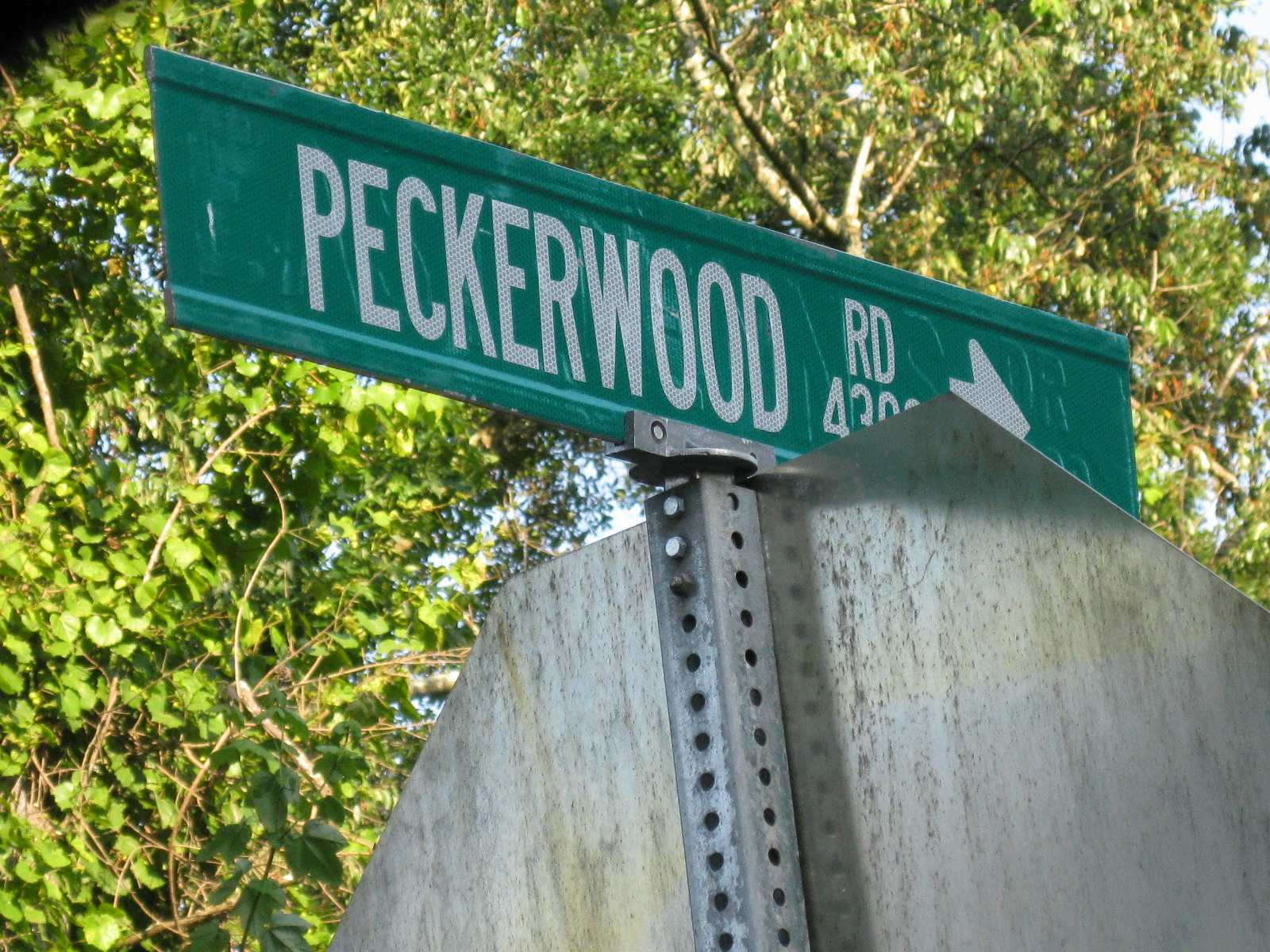In the image, a vibrant, sunlit scene captures the essence of a countryside road. The background is beautifully adorned with an abundance of lush, green trees, their leaves gently rustling in the breeze, while patches of the clear blue sky peek through the canopy. At the forefront stands a green street sign with white lettering that reads "Peckerwood Road," prominently displayed and easily visible. Below the street sign, the backside of a stop sign is noticeable, with its silver metal surface reflecting the sunlight. The edges of the stop sign are darkened, possibly from age or weather exposure, and the metal pole supporting the signs is perforated, displaying several holes along its length. The entire scene is bathed in the warm, golden rays of the sun, highlighting the natural beauty of the leafy surroundings.